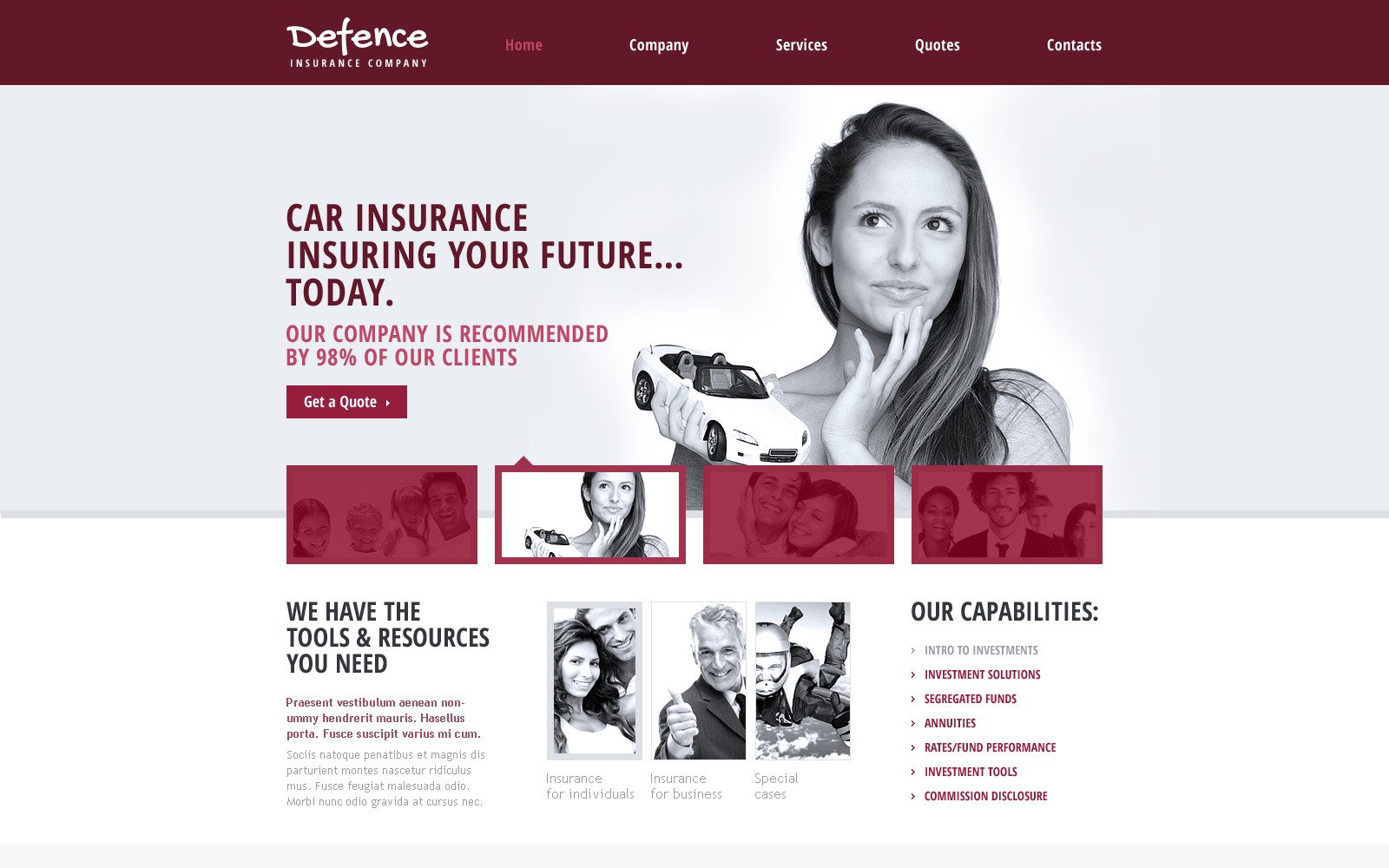The image depicts the homepage of the "Defense Insurance Company" website. In the top-left corner, their logo prominently displays the company name. Adjacent to the logo is a navigation menu with the following options: Home, Company, Services, Quotes, and Contacts. The "Home" tab is highlighted in a pinkish-red color to indicate the current page, contrasting with the white text of the other tabs. The background of this navbar is a deep burgundy stripe.

Immediately below the navbar, a large image carousel features a woman joyfully holding a toy car, gazing into the distance as if lost in thought. To the right of this image, a promotional statement reads: "Car Insurance Your Future Today. Our company is recommended by 98% of our clients." Accompanying this text is a call-to-action button labeled "Get a Quote."

The carousel cycles through four distinct images: 
1. The woman holding a toy car.
2. A happy couple embracing each other, smiling.
3. A man in a suit and tie standing confidently with three people behind him.
4. A cheerful family consisting of a mother, father, and two children being playfully lifted.

Beneath the carousel, a section highlights the company's strengths with the assertion, "We have the tools and resources you need." This area includes three images and a headline titled "Our Capabilities," accompanied by various clickable links to further information.